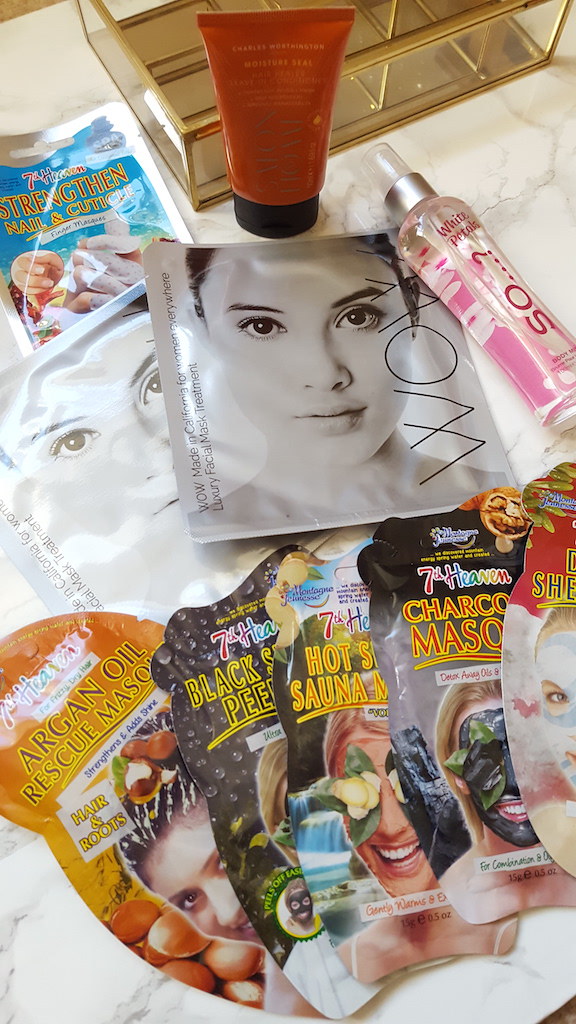In this well-organized display of beauty and personal care products, several items are neatly arranged, each with its own vibrant and eye-catching packaging. At the bottom of the image, five colorful packets of hair masks from the brand 7th Heaven are laid out. These include humorous and descriptive names such as "Hot Sauna," "Charcoal Mask," and "Rescue Mask." Each packet features the brand name prominently at the top and an image of a woman's face near the bottom, making them easily identifiable.

At the center of the display, two monochrome packets resembling magazine covers catch the eye. Each features a woman's face and bold text. One side proudly displays the word "WOW" in large letters, while the other reads "Made in California for Women Everywhere, Luxury Face Mask Treatment," clarifying their actual use as luxurious face masks rather than reading material.

To the right of these face mask packets is a sleek spray bottle labeled "White Petals," indicating it is a body mist. Above this bottle sits a small red plastic container, presumably containing body cream. On the top left, another 7th Heaven product can be seen labeled "Strengthened Nail and Cuticle Treatment," aimed at enhancing nail care.

Crowning the display at the very top is an elegant, golden-colored box, likely intended for storing trinkets or jewelry, adding a touch of sophistication to the overall arrangement. This beautifully staged assortment of beauty and personal care items showcases a range of treatments designed to pamper and enhance various aspects of personal grooming.